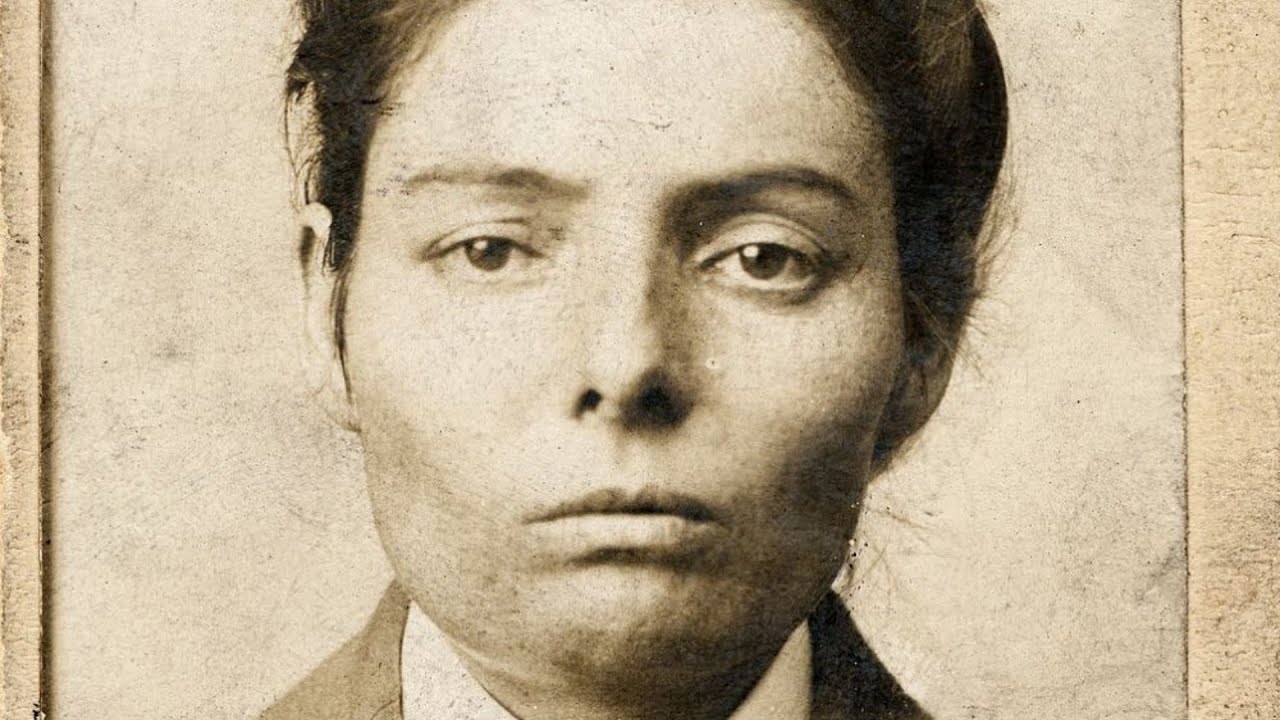In this close-up, sepia-toned image, we see an androgynous individual with dark, pulled-back hair, potentially in a bun, which frame their serious expression. The photograph, which appears aged, is cropped just above the forehead and below the chin, revealing only the top part of their torso. The person's eyes are dark and heavily hooded, with slightly downcast eyelids, giving them a somber, unsmiling demeanor. They have thin eyebrows, large eyes, a small nose, and medium-sized ears. The individual is wearing a white-collared shirt under a darker jacket, which is discernible by the visible top of the apparel. The background is a simple, light sepia tone with a light brown strip along the right side. The overall composition and subdued expression suggest a feeling of sadness or solemnity.